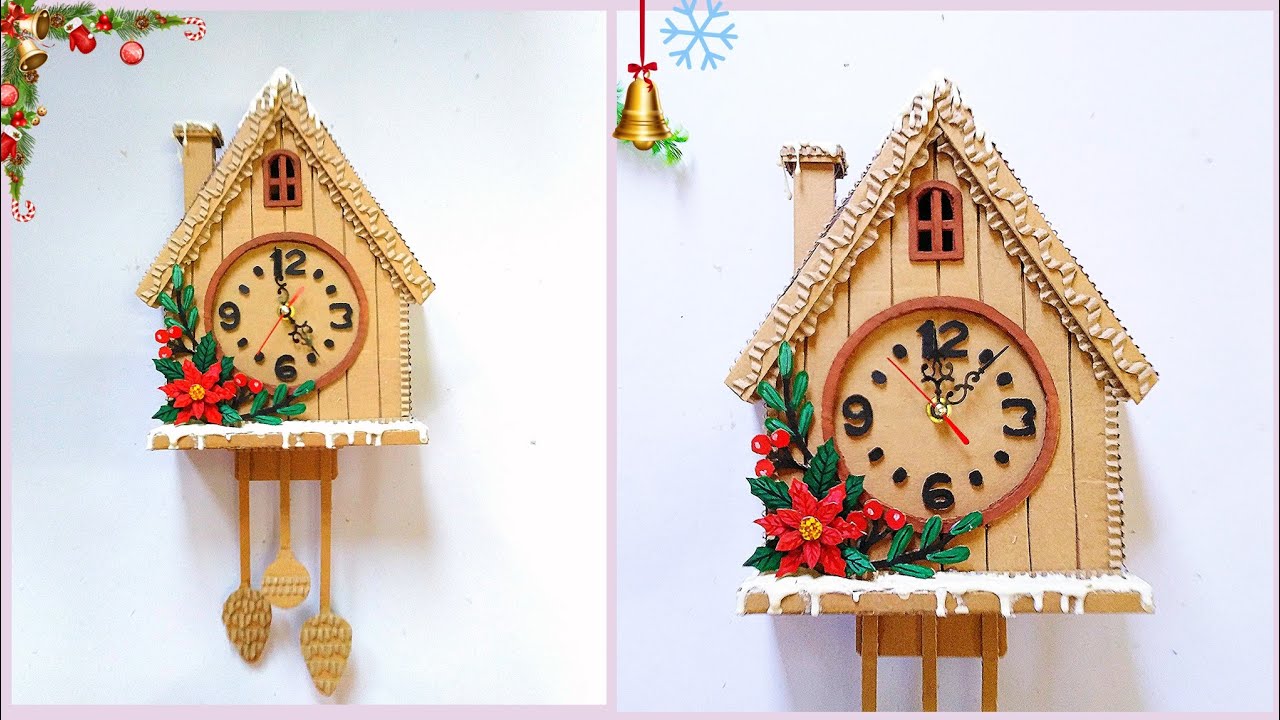The image shows two side-by-side photographs of a handmade, Christmas-themed cuckoo clock. The left image presents a zoomed-out view, while the right offers a close-up. The clock is crafted from a light tan material, resembling cardboard or balsa wood, and is designed to look like a Swiss-style house with a peaked roof and a chimney, both dusted with fake snow that simulates icing.

In the left image, the clock face shows the time as just before 4 p.m., decorated with black Arabic numerals (12, 3, 6, 9) and black dots marking the other hours. Three pine cone-shaped pendulums hang from the base of the clock. A poinsettia with greenery adorns the bottom left, while Christmas decorations, including bells, ornaments, and a candy cane, are illustrated in the top left corner of the image.

The right image is a close-up of the same clock, now showing the time as 12:05. The close-up highlights a golden bell with a blue snowflake hanging in the top left corner. This image captures more detail of the clock’s intricate design, including its small arched window at the top peak, possibly where a cuckoo bird would emerge, if functional. Both images have a white, slightly textured background, adding a clean, festive atmosphere to the setup.